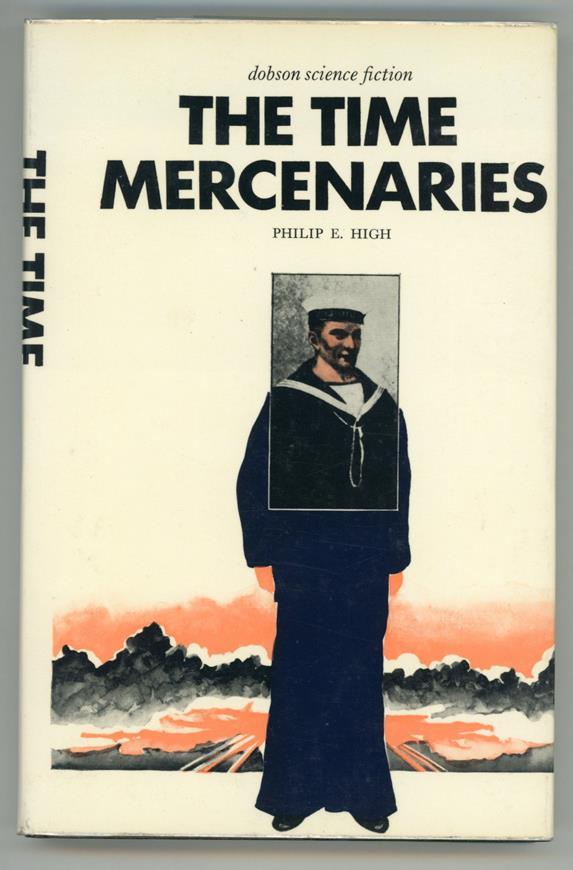The cover of the book "The Time Mercenaries" by Philip E. High, published by Dobson Science Fiction, features a detailed illustration of a military sailor. The sailor is depicted in a navy blue uniform with white piping, a distinctive white sailor hat with a black band, and black shoes. He stands on a white platform or ground, with a backdrop of abstract, smeared orange and gray imagery that includes mountains, a road, and trees rendered in a pencil-like style. The book has a gray cover with a darker gray spine that also bears the title "The Time" and the author's name in black text. The overall design suggests a vintage or older publication, sitting possibly on a table or stand.